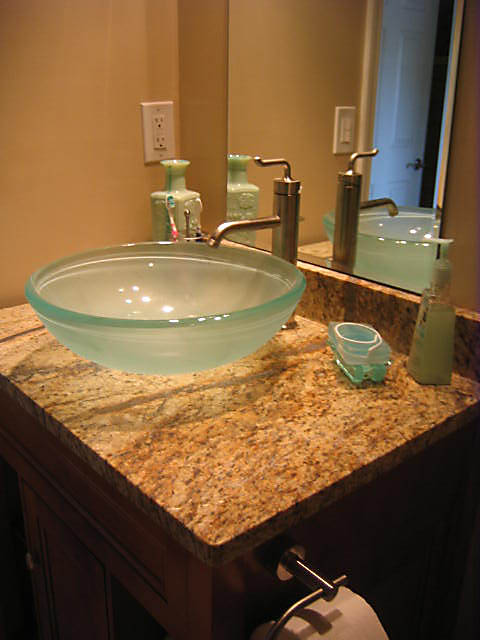A luxurious bathroom featuring a sophisticated vanity setup: The bathroom walls are painted in a calming light brown-tan hue, providing a warm backdrop. The vanity is topped with an elegant brownish-red granite surface, which is complemented by a matching granite backsplash. Mounted above the vanity is a large, frameless wall mirror that spans the width, reflecting the space's refined aesthetic.

The centerpiece of the vanity is a striking, wide but shallow glass bowl sink. The bowl is translucent with a faint green or aqua tint, adding a subtle pop of color. Above it, a sleek, upright, single-knob faucet delivers water into the bowl, whose elegant design is mirrored in the reflection behind it.

To the left, a white power outlet is visible on the wall, just above a decorative green milk glass bottle that adds a touch of vintage charm. Adjacent to it, a caddy holds two toothbrushes, keeping everyday essentials within easy reach.

On the right-hand side of the vanity, there's a stylish liquid soap dispenser. In front of the dispenser, an enigmatic object, possibly made of a similar green glass, sits, its exact purpose unclear, yet undeniably adding to the overall aesthetic appeal. The blend of materials, colors, and functionality create a bathroom that is both practical and exquisitely designed.